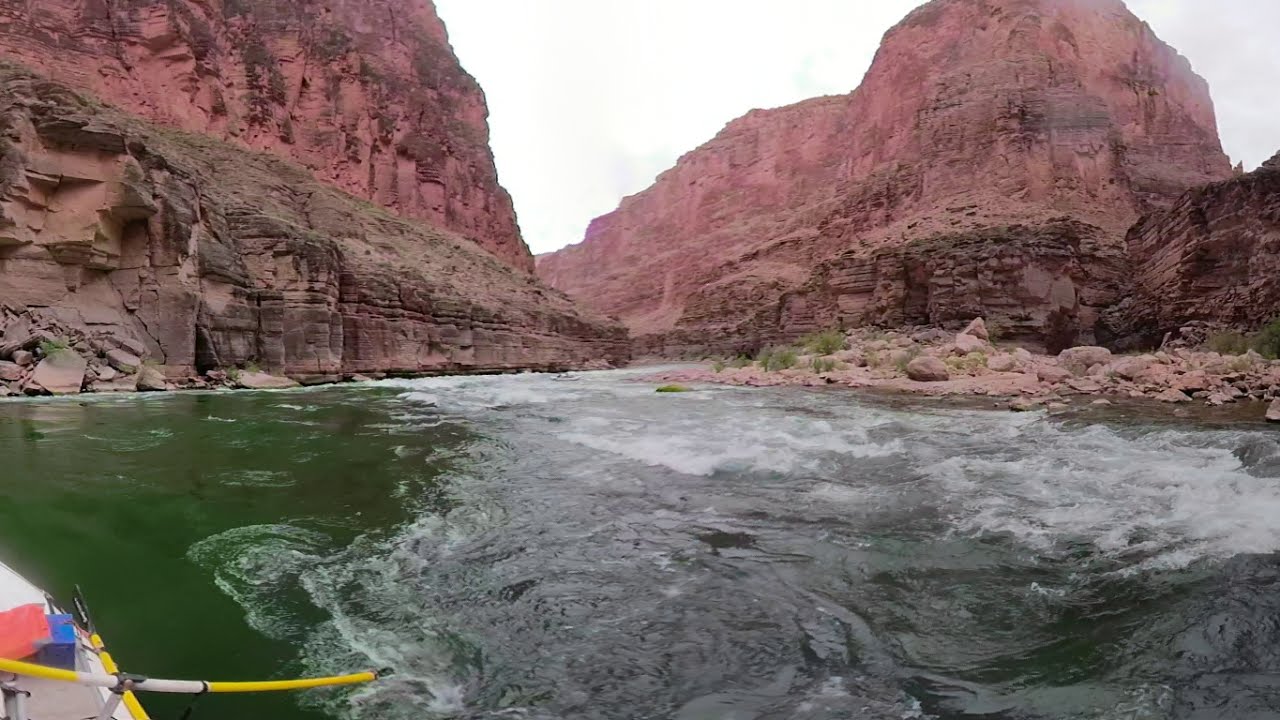The image depicts a thrilling scene of rafting down a tumultuous river, likely part of the Colorado River, nestled between towering, reddish-brown canyon walls, reminiscent of the Grand Canyon's majestic landscape. At the very bottom left of the frame, a yellow and white oar can be seen extending into the water from the corner of a raft, suggesting movement through moderate white-water rapids classified as Class II. The river, which appears somewhat murky and green, bends to the left, directing the raft away from the rocky shores on either side. The canyon walls, eroded over time, rise steeply with visible sediment layers, creating a dramatic backdrop. The wide-angle lens captures the expansive scene with a slight distortion, emphasizing the rough waters and rugged terrain. The sky above is bright, indicating a clear day, despite some overcast areas allowing sunlight to peek through. No people are visible in the photo, placing focus on the dynamic interplay between the river and the canyon.